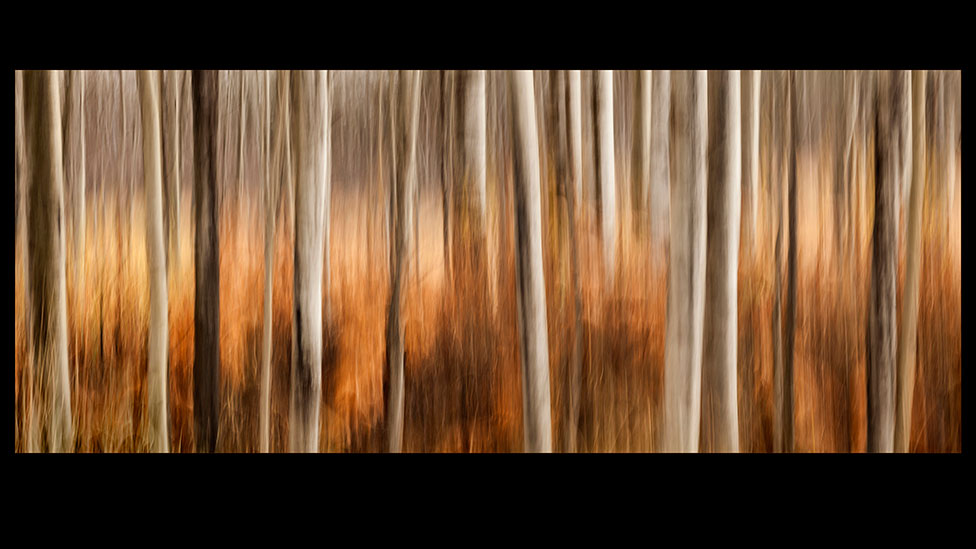This image is an abstract, nature-inspired painting depicting a dense forest scene. In the center of a completely black background, the rectangular artwork features vertically oriented tree trunks stretching from left to right. These trunks vary in shade and hue, ranging from white to taupe, and are highlighted by earthy tones of brown, orange, and rusty yellow. The lighting and shading create a sense of depth and form, with no bright or vivid colors present. Surrounding the trees, the ground is depicted with overgrown dried grass and brambles, contributing to the wilderness feel of the piece. The image has no text and is purely artistic, capturing the essence of a wooded area with a focus on the earthy, naturistic palette.